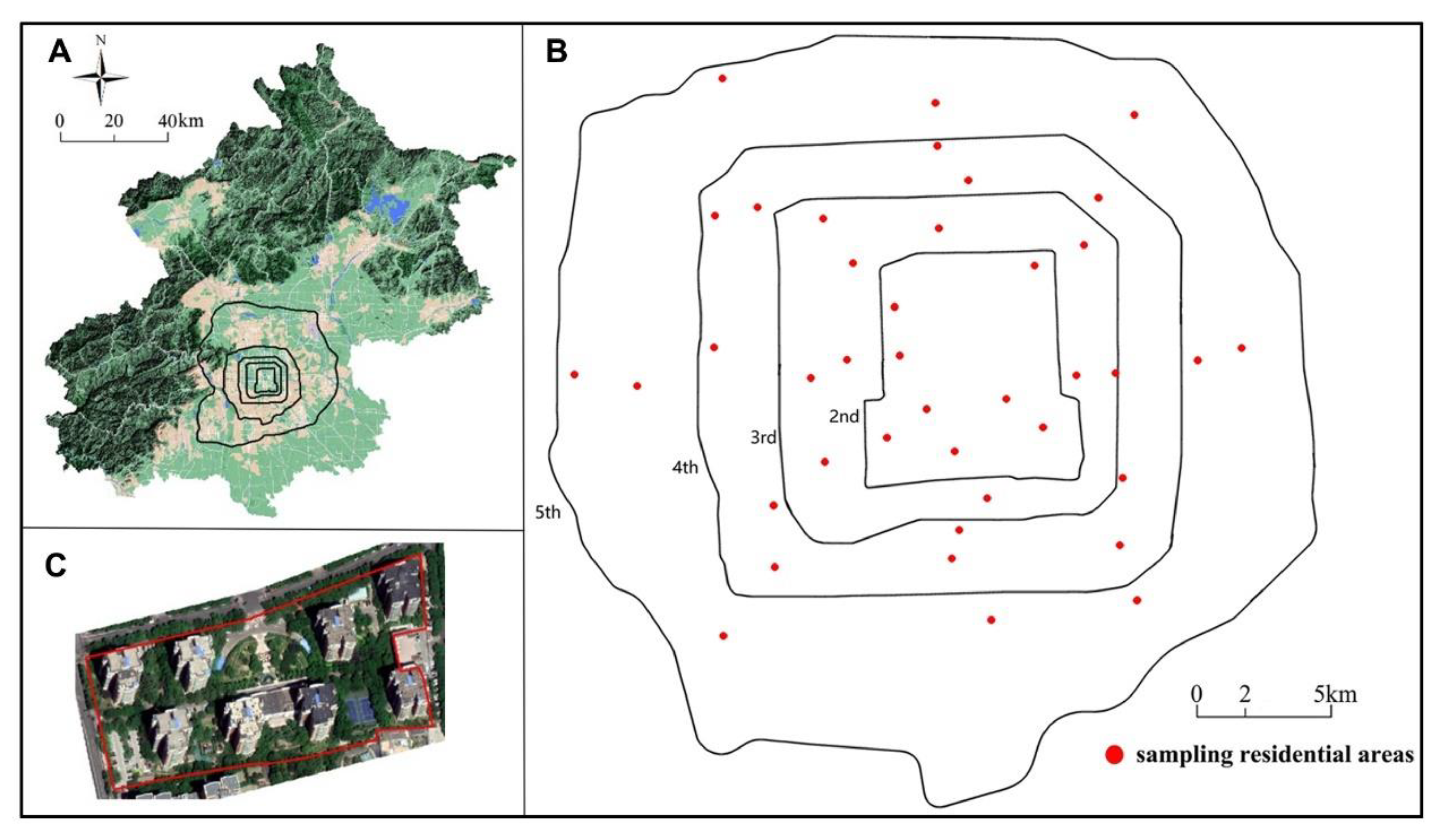This detailed image is divided into three labeled sections: A, B, and C. The top left segment, marked A, presents a topographical map featuring a letter A, a north-pointing compass, and a scale bar ranging from 0 to 40 kilometers. This map outlines a landmass with various regions colored differently, including patches of lighter green, blue, and brown, as well as some darker, partially erased areas.

The largest section, labeled B and situated to the right of the image, contains a line diagram with overlapping concentric shapes in various colors. These shapes are labeled as "fifth," "fourth," "third," and "second," decreasing in size from the outermost to the innermost. Red dots interspersed between these shapes denote residential sampling areas, with a scale bar indicating distances of 0, 2, and 5 kilometers.

At the bottom left, the section labeled C shows an aerial photograph of a rectangular piece of land, slightly angled, and bordered with a red outline. This image details a cluster of six houses surrounded by green trees, illustrating the residential areas mentioned in section B.